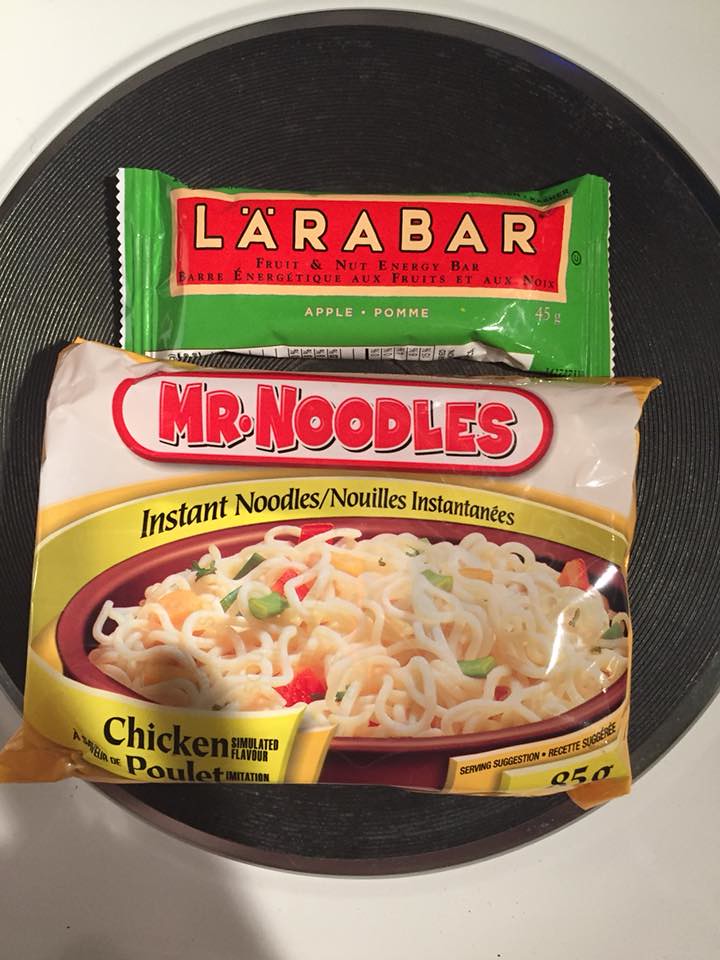This image features a clean white background with a centrally placed black circular object, which could be a plate, placemat, or stove burner. On top of this black surface are two food items: a Larabar fruit and nut energy bar and a packet of Mr. Noodles instant noodles. 

The Larabar is positioned above the noodles and has a green plastic wrapper with a red rectangle that contains the brand name "Larabar" in yellow text. Below, it reads "Fruit and Nut Energy Bar" and "Apple" alongside some French writing. 

Beneath the Larabar is a yellow and white packet labeled "Mr. Noodles" in red text, indicating it contains chicken flavor instant noodles. The packet features an image of a bowl filled with noodles, along with some finely chopped red and green bell peppers, although these ingredients are likely just for the illustration. The words "Instant Noodles" are displayed around the bowl image, along with serving suggestions and additional French text.

Together, these items form a visually interesting composition focused on commonly consumed prepared food products.